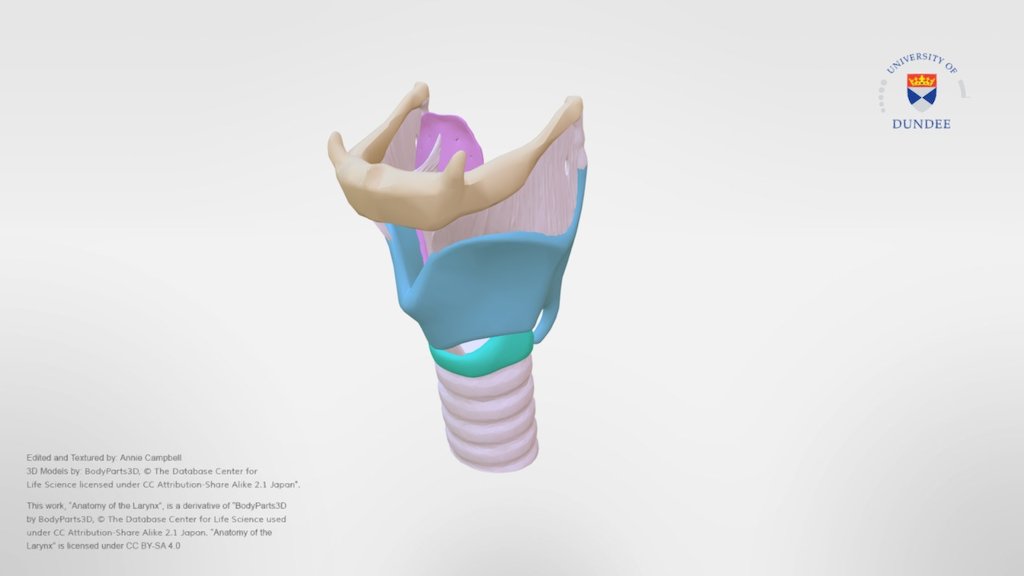This image is a detailed 3D model representation of the anatomy of the larynx, set against a white background. At the center, the prominent feature is a realistic depiction of a lower jaw bone, under which lies a blue 3D model of the neck and spine, with the spine rendered in a peach hue. The different parts of the larynx in the illustration are distinguished by various colors, utilizing around five distinct shades.

In the top right corner of the image, there is a circular emblem. The top of this circle features blue text reading "University of." Centrally positioned within the circle is a shield emblem adorned with a red top containing a yellow crown and two blue triangles beneath it. The bottom portion of the circle contains blue text that reads "Dundee."

In the bottom left corner, there is a small gray text attribution: "Edited and textured by Anne Campbell. 3D models by BodyParts3D at the Database Center for Lifesize License under CC Attribution Share Alike 2.1 Japan." Below this, it further explains, "This work, Anatomy of the Larynx, is a derivative of BodyParts3D by BodyParts3D Incorporated. Larynx is licensed under CC BY SA 4.0."